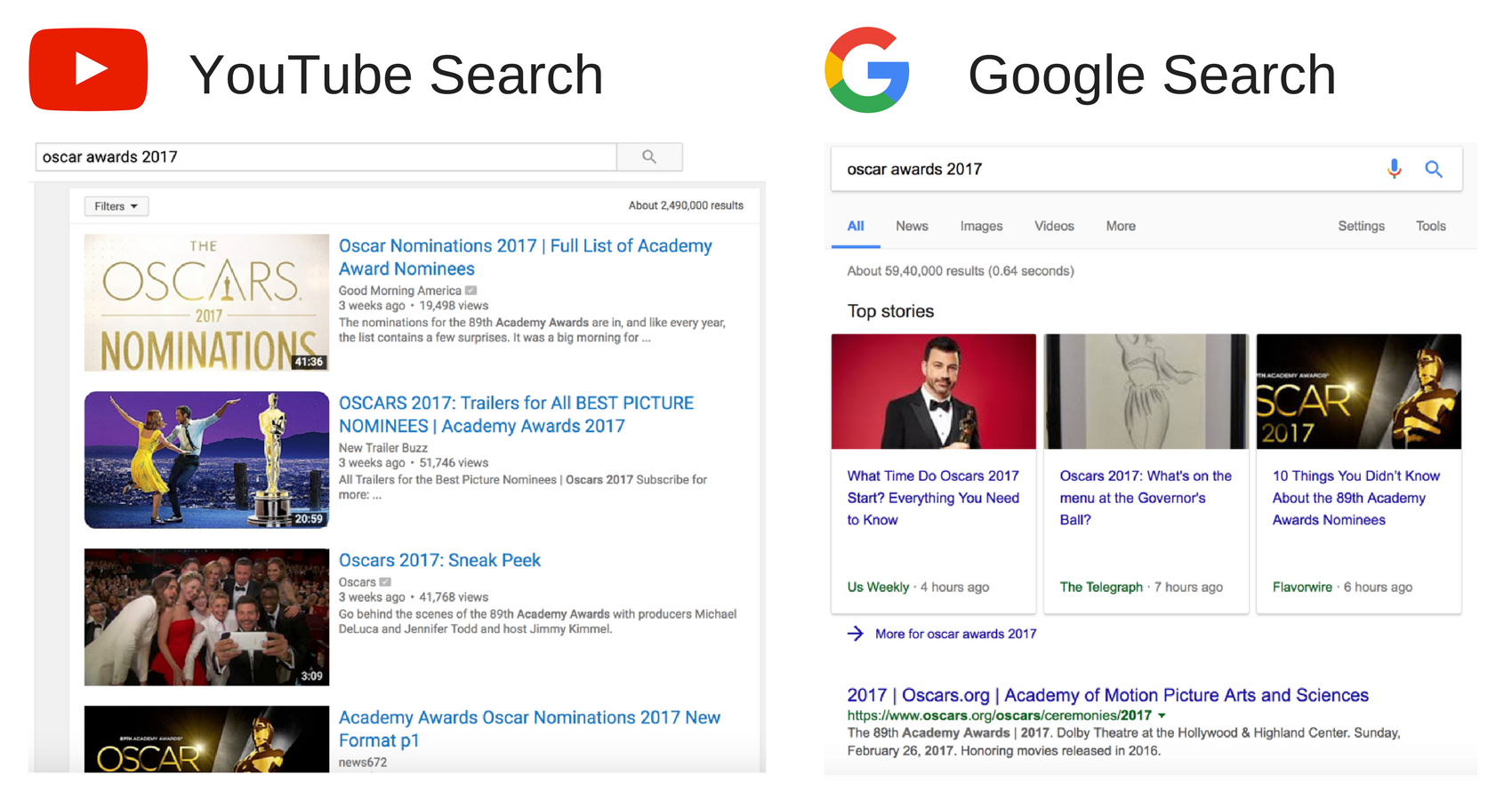This image is a split-screen comparison showcasing search results for "Oscar Awards 2017" from YouTube and Google. On the left side, the YouTube search results are displayed. The search query "Oscar Awards 2017" reveals a list of video content, including a 41-minute clip titled "Oscar Nominations 2017: Full List of Academy Award Nominees" from Good Morning America, a "2017 Best Picture Nominees Trailer" by New Trailer Buzz, and a sneak peek video from the official Oscars YouTube channel. Another video, "Academy Awards: Oscar Nominations 2017 New Format," is also visible in the list.

The right side of the image shows Google search results for the same query. The search is performed under the "All" tab, presenting top stories such as "What time do the Oscars 2017 start?" and "Everything You Need to Know: Oscars 2017." Additional articles include "What's on the Menu at the Governor's Ball" and "10 Things You Didn't Know About the 89th Academy Award Nominees." The search results also include a link to the official Oscars website, Oscars.org, which discusses the 89th Academy Awards.

The image effectively demonstrates the differences in search results between YouTube and Google for the same event, highlighting the types of content each platform offers.